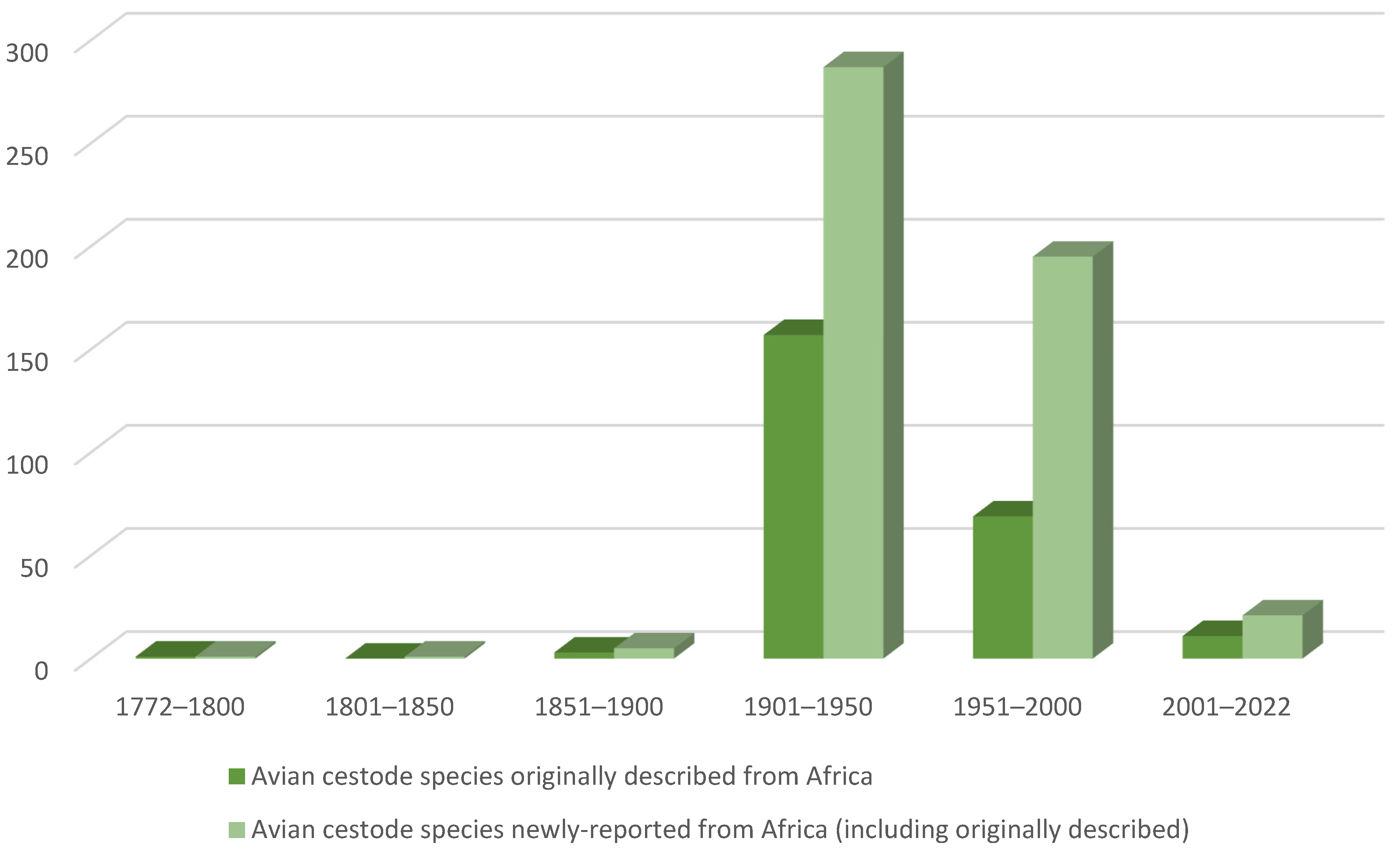The image displays a detailed vertical bar graph representing the counts of avian cestoid species described and reported from Africa over various time periods. The vertical axis is labeled from 0 to 300 in increments of 50, while the horizontal axis lists the periods 1772 to 1800, 1801 to 1850, 1851 to 1900, 1901 to 1950, 1951 to 2000, and 2001 to 2022. Each period is represented by two bars: a dark green bar for "avian cestoid species originally described from Africa" and a light green bar for "avian cestoid species newly reported from Africa, including originally described." 

In the periods 1772 to 1800, 1801 to 1850, and 1851 to 1900, both bars remain at zero. The period of 1901 to 1950 shows a significant rise, with the dark green bar reaching 150 and the light green bar approaching 275. For 1951 to 2000, the dark green bar drops to just above 50, while the light green bar falls to just below 200. In the final period, 2001 to 2022, both bars decrease substantially, with the dark green bar slightly surpassing 20 and the light green bar reaching around 30.

The legend below the graph clarifies the difference between the dark green and light green bars, ensuring clear understanding of the data presented.